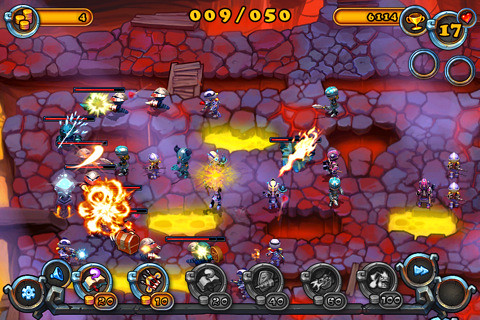This is a vibrant, detailed screenshot from a mobile video game that features a horizontal rectangular surface. The backdrop showcases a colorful, cartoonishly drawn volcanic terrain with purple and red rocky structures interspersed with pits of yellow lava. The setting appears to be the site of an intense battle, with various tiny blue enemies, noticeable explosions, and fiery projectiles illuminating the scene. The top of the screen displays several oblong orange lines with white numbers and a prominent yellow "009/050" indicator in the center. Additional HUD elements include a money symbol with a "4" in the upper left-hand corner, and a "6114" with a crown and a "17" on the right. The bottom of the screen is lined with a series of round, clickable icons or buttons essential for gameplay. The vibrant, simplistic art style and bright, contrasting colors contribute to a lively and chaotic battlefield atmosphere, enhanced by large purple figures at the edges emitting yellow flames and one figure on the right sporting reddish hair and a long red nose.